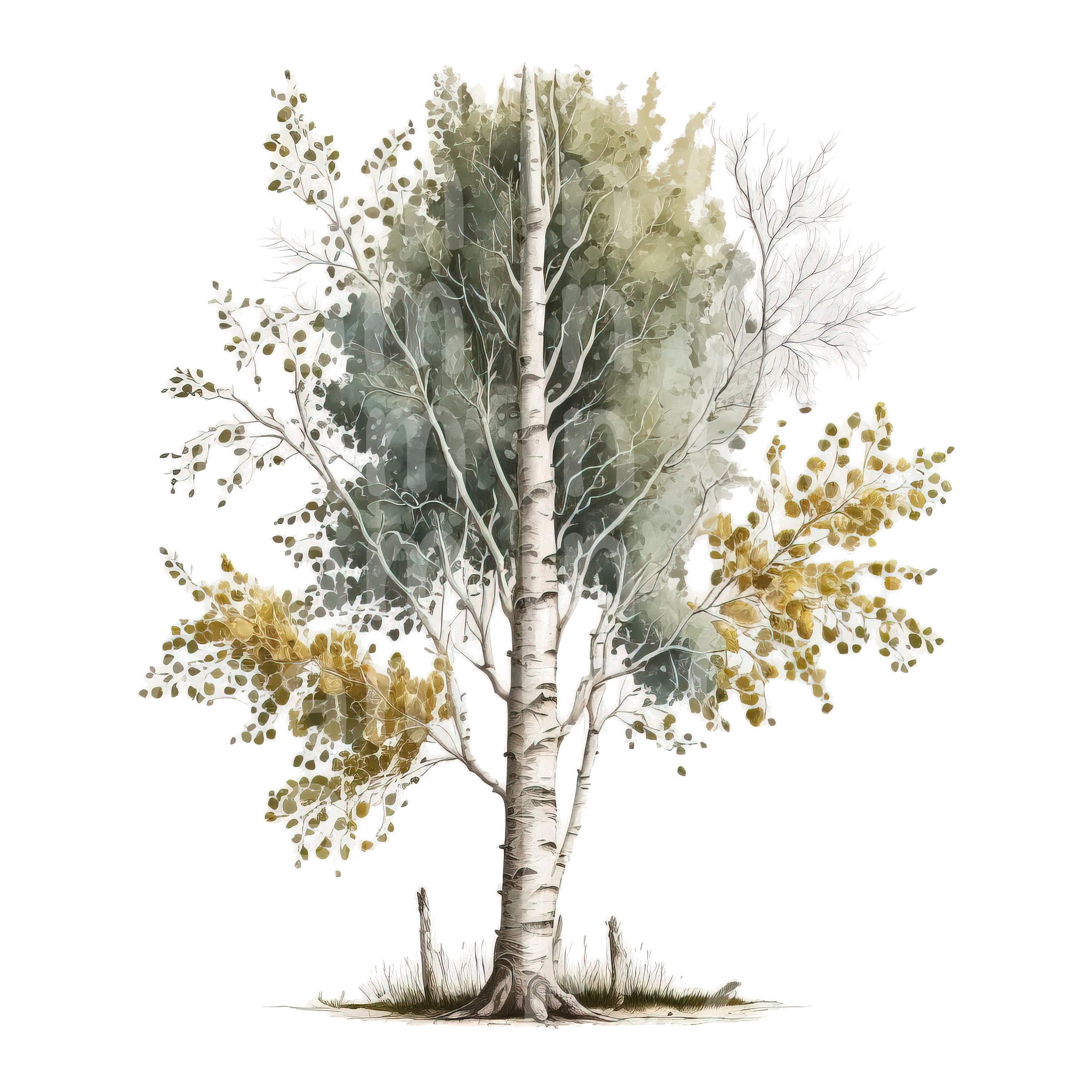This image showcases a detailed watercolor painting of a birch tree set against a completely white background, devoid of any frame or additional elements. The tree is depicted with a striking white trunk, characterized by its flaky, paper-like texture and brown markings. Numerous branches extend from the trunk, some of which are barren, while others flourish with foliage. The leaves on the tree vary in color and type; some are yellow and round, while others are green, forming a central plume near the top where individual leaf details blend into shades of dark to light green. At the base of the tree, several white roots visibly plunge into the ground, surrounded by patches of grass that range in color from green to dark brown. Additionally, small wooden outshoots or posts are seen near the bottom of the tree, enhancing the naturalistic detail of the scene. The painting captures the seasonal transition of the tree with its mix of lush green, sparse green, and golden yellow leaves, all set against the stark simplicity of the white background.